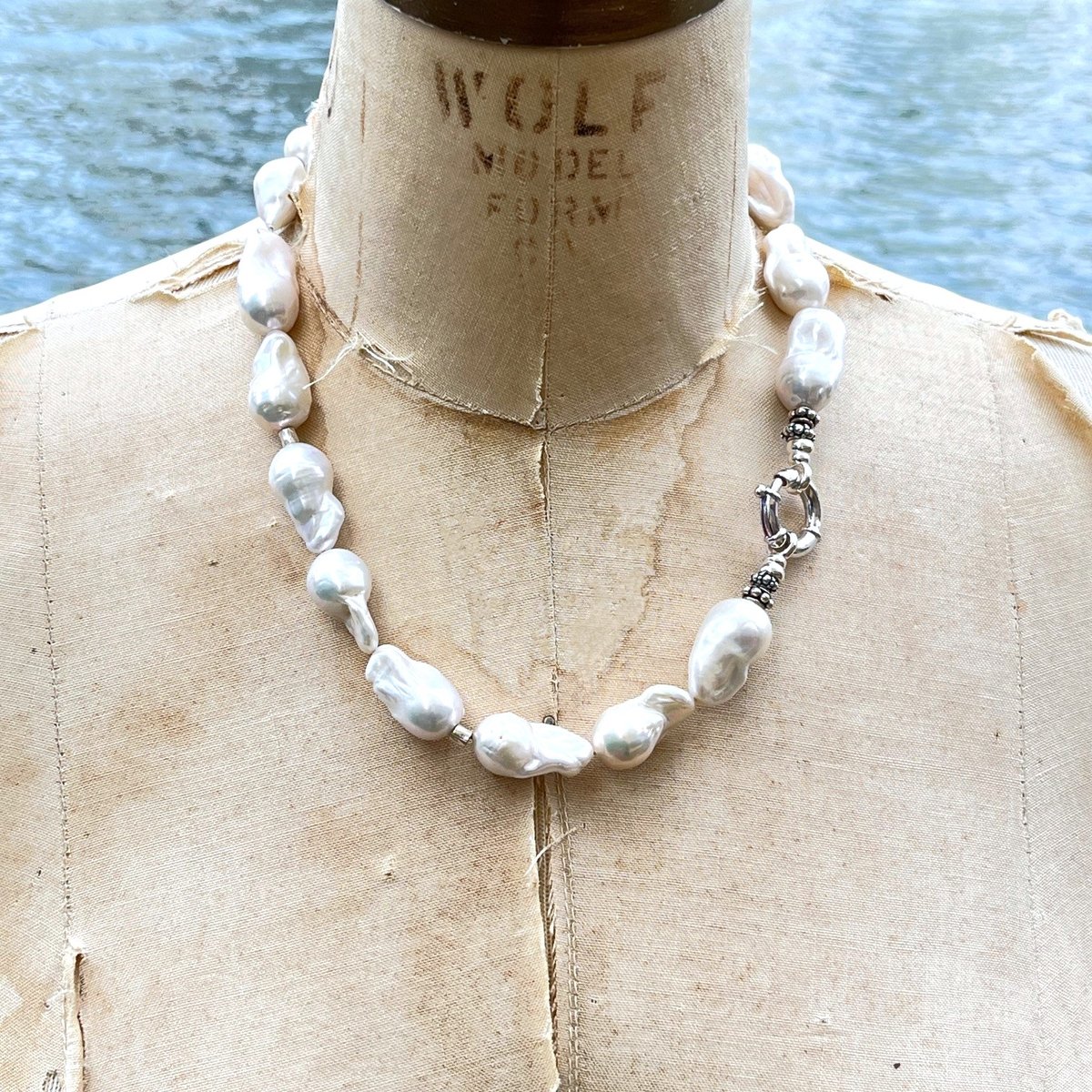The photograph showcases a highly aged and tattered mannequin draped in a beige, stained fabric, marked with the words "Wolf Model" around its neck. The mannequin's surface appears largely damaged with visible signs of wear, including dust, water stains, and some broken portions. Adorning its neck is a striking, imperfect pearl necklace comprised of irregularly shaped, iridescent white stones that glisten with a metallic sheen. These pearlescent elements are strung together with a combination of plastic string and metal chains, and the right side of the necklace features a noticeable silver or metal attachment. The backdrop of the image hints at an outdoor setting, potentially with a body of water or a blue building wall adding to the scene's overall vintage and weathered aesthetic.